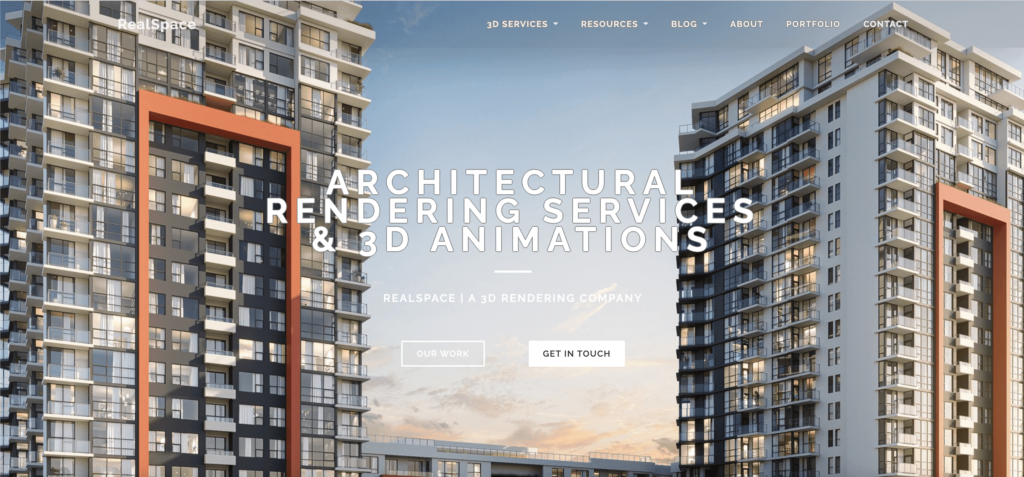The screenshot depicts a detailed architectural rendering of an urban skyline, featuring two prominent tall buildings that appear to be residential apartments. Adjacent to these is a third, significantly shorter building. The sky is filled with clouds exhibiting shades of orange and gray, imparting a dramatic and somewhat serene atmosphere to the scene.

Overlaying this image is clear white text that reads "Architectural Rendering Services and 3D Animations," indicating the professional services offered by "RealSpace," a 3D rendering company. Two interactive buttons are prominently displayed: one in a gray rectangle labeled "Our Work" and another in a white rectangle with the text "Get in Touch."

At the top of the screenshot, a navigation menu lists several options: "3D Services," "Resources," "Blog," "About," "Portfolio," and "Contact." Notably, each of the first three menu options features a downward-pointing triangle, suggesting the presence of dropdown menus for further navigation.